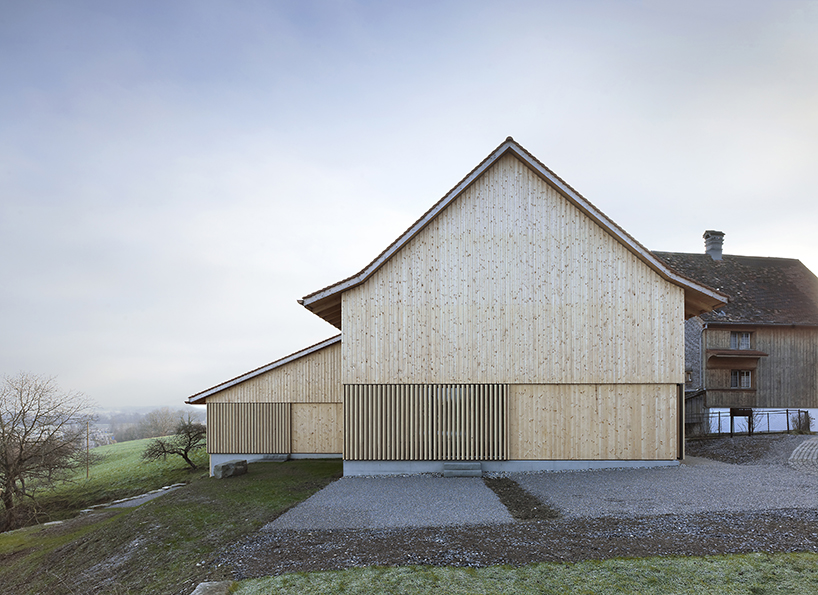Perched on a grassy hill in a remote area, a very large house stands majestically against a backdrop of blue skies with scattered white clouds. The house appears to be at least three stories high and features a striking architectural style with natural wood planks aligned vertically. The façade of the structure showcases a mix of light brown, black, and darker brown tones, creating a visually appealing contrast.

On the left, there is a barn-like extension with a triangular, pointed roof that lacks windows or doors, suggesting it might still be under construction. This section is clad in natural, unstained wooden boards. Adjacent to this, the main building features a beautiful slanted black roof with white eaves that extend downward. The light wood of the structure is perfectly maintained, adding to its stunning appearance.

In the front, patches of gray gravel interspersed with brown spots cover the ground, leading towards the building. A sliver of green grass runs from right to left, thinning out towards the left side of the image. This leads to a hill that slopes gently downward, offering a panoramic view of the distant landscape, which fades into a valley with trees and hints of additional buildings.

A small tree, likely in early spring, stands out without leaves, indicating the seasonal transition. On the right side of the house, another structure with a brown roof and possibly a small balcony is visible, with windows bordered in white. A road edges the scene, enhancing the resort-like quality of the location. Overall, the image captures a serene, expansive setting with a beautifully detailed, rustic house as the focal point.